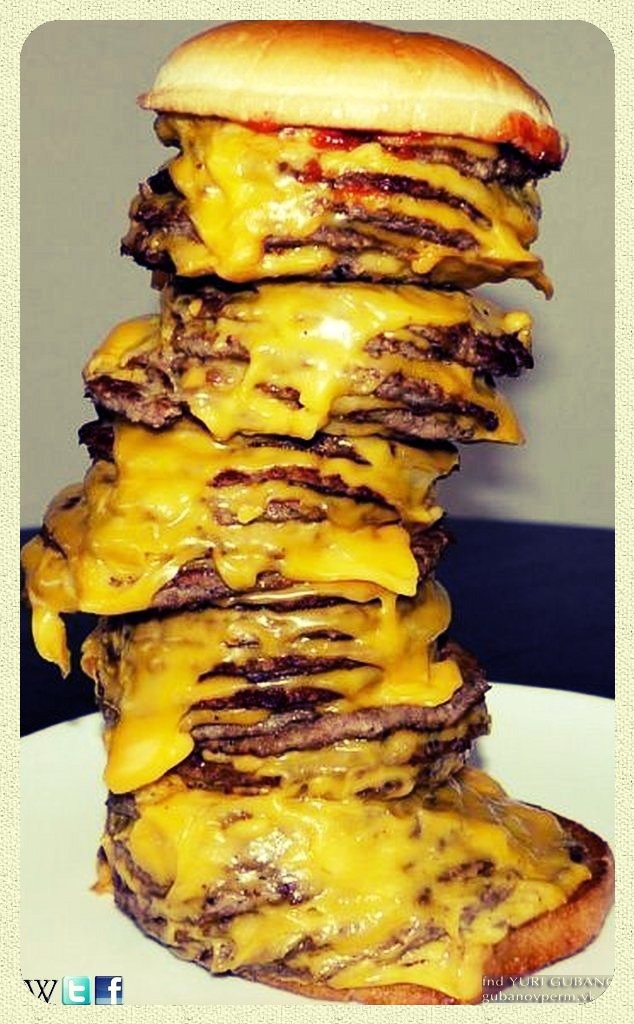This photograph showcases an absurdly tall and outrageous cheeseburger against a beige and gray backdrop. The image captures a monumental stack of cheeseburgers, comprising approximately 27 to 33 layers of thin hamburger patties, each generously slathered with melted cheddar cheese. The towering burger rests on a white plate, with a toasted bottom bun at the base and a slightly askew top bun crowned with a smear of ketchup. The cheese oozes down the sides, adding to the visual overload. The setup includes a trim of light cream canvas and a noticeable strip of black against the wall behind it. Social media logos are visible in the lower corners, along with the tag "FND Yuri Gubanovperm.VK." Overall, the cheeseburger's excessive height and gooey cheese make it a spectacle that's both tantalizing and overwhelming.